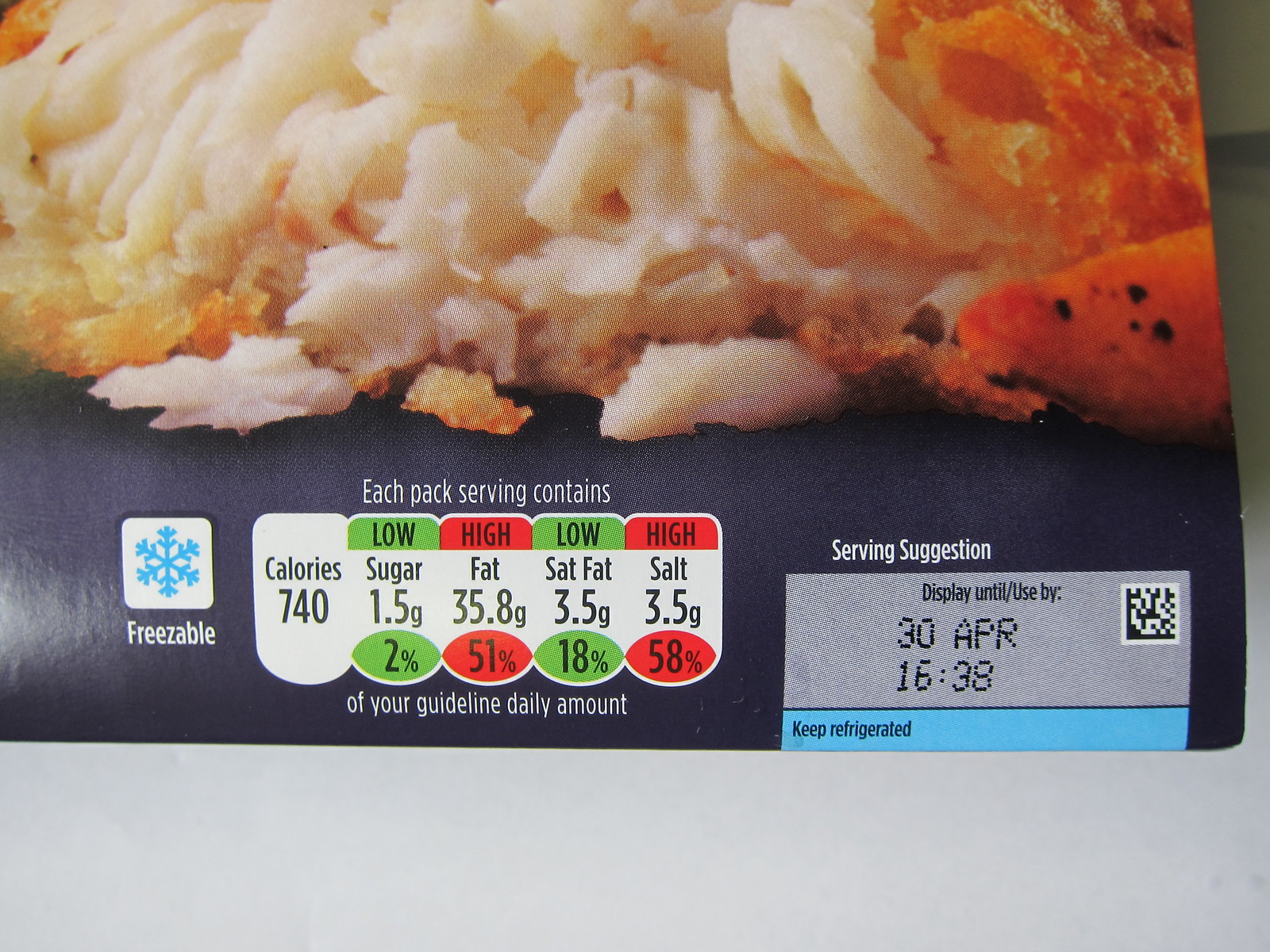This photograph captures the bottom right corner of packaged, pre-made, reheatable food. The visible portion of the packaging showcases an image that might be hash browns or breaded fish, distinguished by a golden-brown texture to the top right and a white portion that could be potatoes or cheese in the center. To the bottom left, a blue snowflake icon signifies that the product is freezable, and nearby, the nutrition information reads: 740 calories, low sugar at 1.5 grams (2%), high fat at 35.8 grams (51%), low saturated fat at 3.5 grams (18%), and high salt at 3.5 grams (58%). The packaging is color-coded with green for low content and red for high content of nutrients. On the bottom right, it states "serving suggestion" and "display until used by April 30" alongside a barcode, with the timestamp of 16:38.